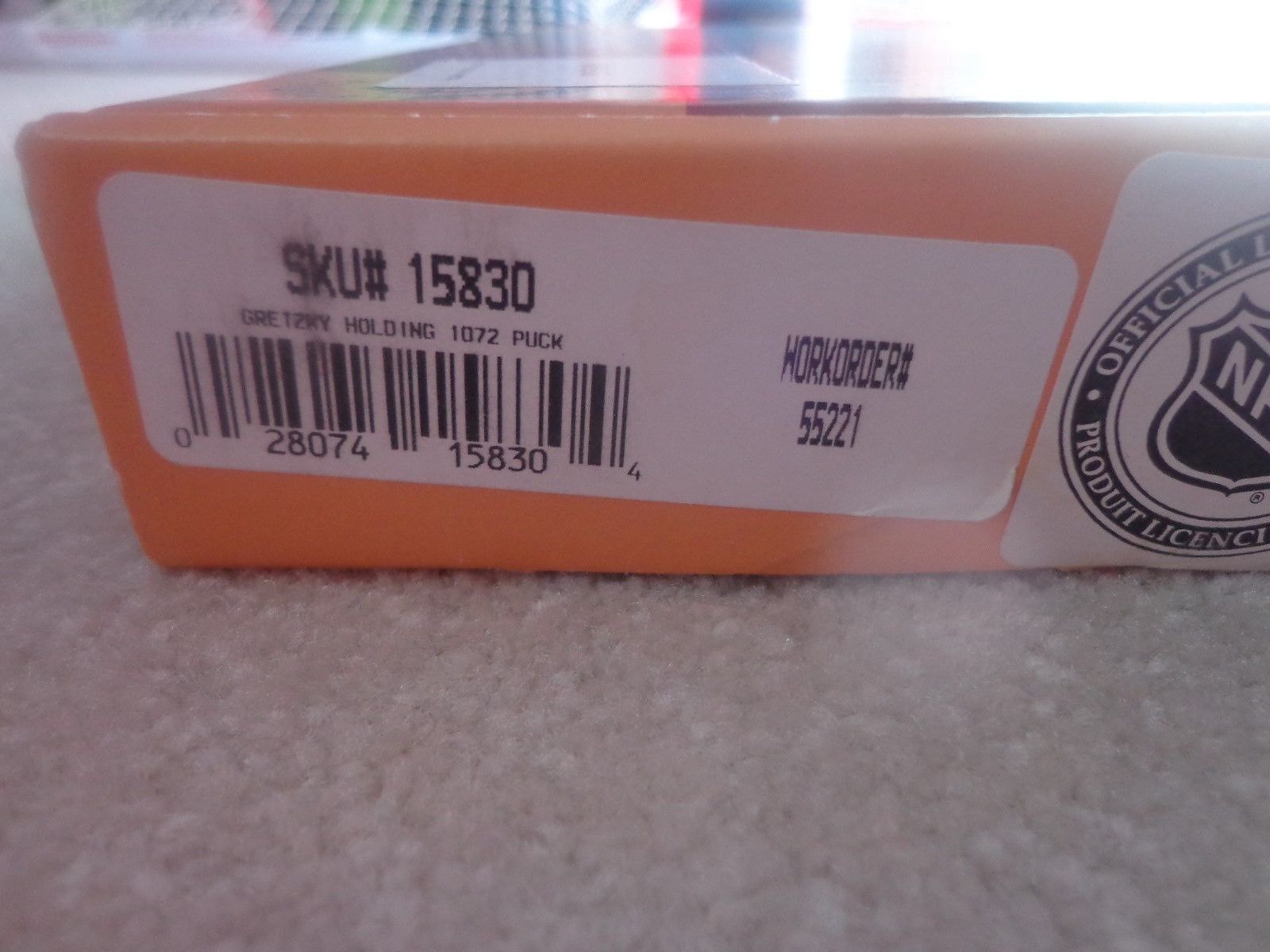The image is a zoomed-in color photograph focusing on the bottom of an orange package lying flat, possibly on a white carpet. The main feature is a white label displaying various identification details including two barcodes and a SKU number (15830). The text includes "Gretzky Holden 1072 puck" alongside a work order number (55221). Part of the packaging reveals an official product license, though it's partially cut off and spelled "P-R-O-D-U-I-T license". To the right, there's a glimpse of what appears to be the NHL logo with truncated letters "N-H". Due to the details such as the Gretzky reference and official licensing, it can be inferred that the item is sports-related, possibly a puck associated with Wayne Gretzky.